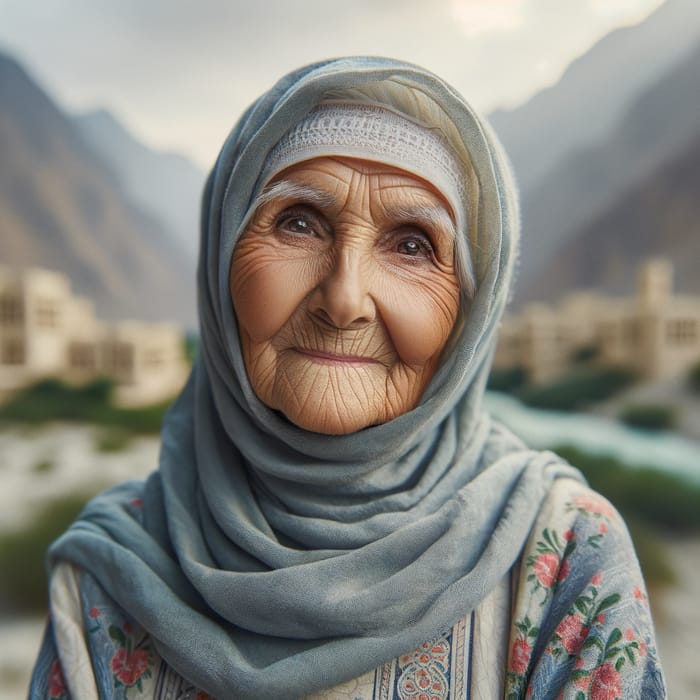The close-up image features an elderly woman wearing traditional attire, captured with intricate detail. She dons a light blue dress adorned with pink flowers and a matching light blue scarf that drapes over her head and shoulders. Underneath the scarf, a white bonnet is visible. Her long gray eyebrows and deep brown eyes contrast with her aged, wrinkled face, reflecting the spirit of a younger woman within. The woman is smiling warmly at the viewer. The digital artwork highlights the smooth texture of her face despite the wrinkles. The background is blurry but reveals a valley setting with tall, steep mountains and several light tan buildings, evoking a Middle Eastern ambiance. The cloudy, overcast sky adds to the depth of the scene, enhancing the sense of realism in this AI-generated image.